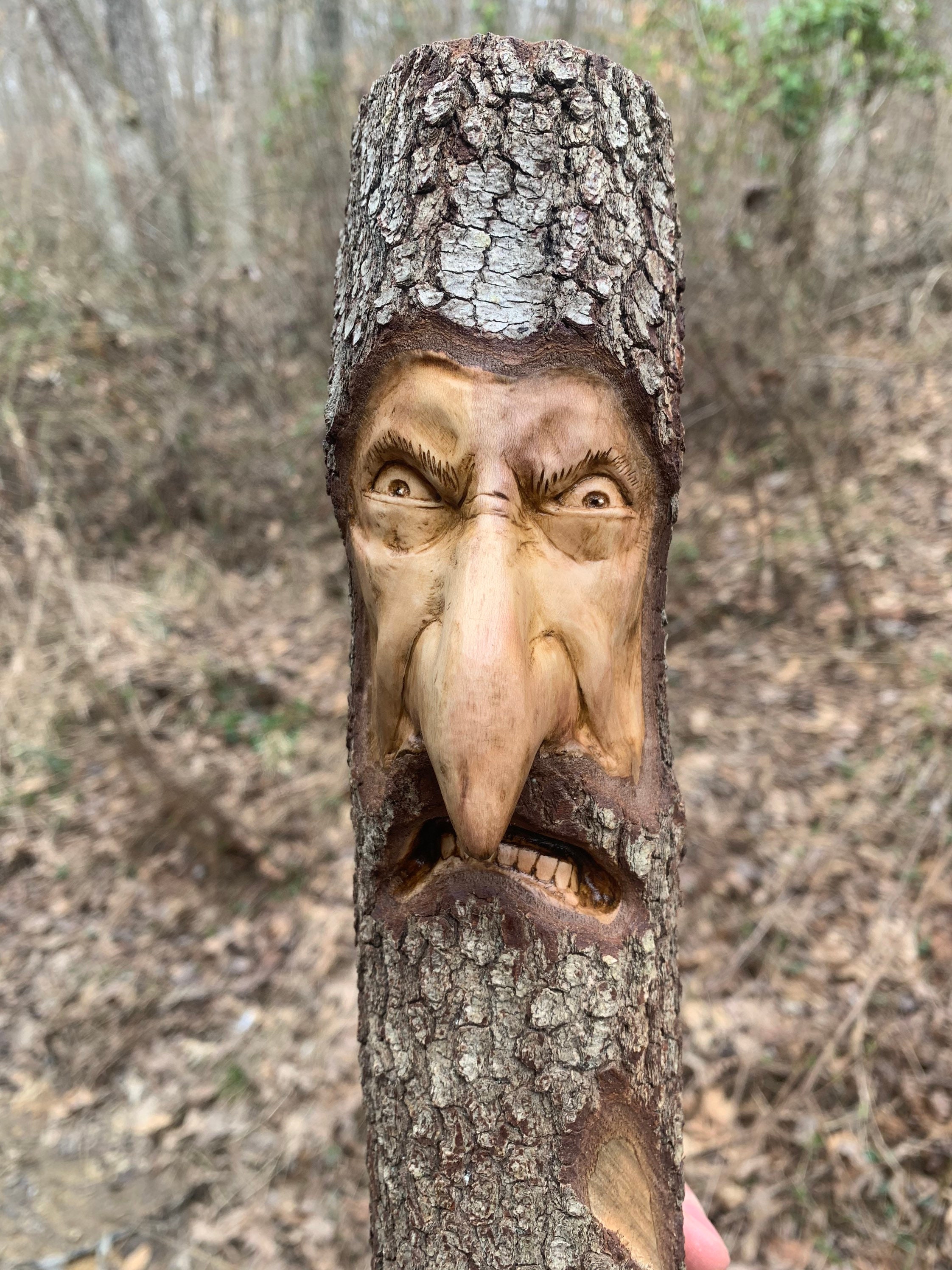In the center of the image, a menacing face is intricately carved into a narrow, tree trunk or wooden log, resembling a troll or a character from Monty Python and the Holy Grail. This carved face portrays a terrifying expression with ominous, angry eyes that are wide open but have small pupils, and scrunched, arched eyebrows. The most distinctive feature is the exaggerated, very long, and pointed hook nose that extends all the way down to his open mouth, displaying grimacing teeth. The carving is highly detailed, presenting a blend of both realistic and cartoon-esque qualities. Surrounding the carved section, the top and bottom parts of the tree trunk retain their natural bark, blending organically into the wooden log. In the blurred background, the forest floor is visible with leaves and twigs strewn about, indicating a gray day with the forest and tree trunks depicted in shades of gray, adding a contrasting backdrop to the light-colored carved face. There's also a subtle hint of a thumb, suggesting someone might be holding the carved log in place.